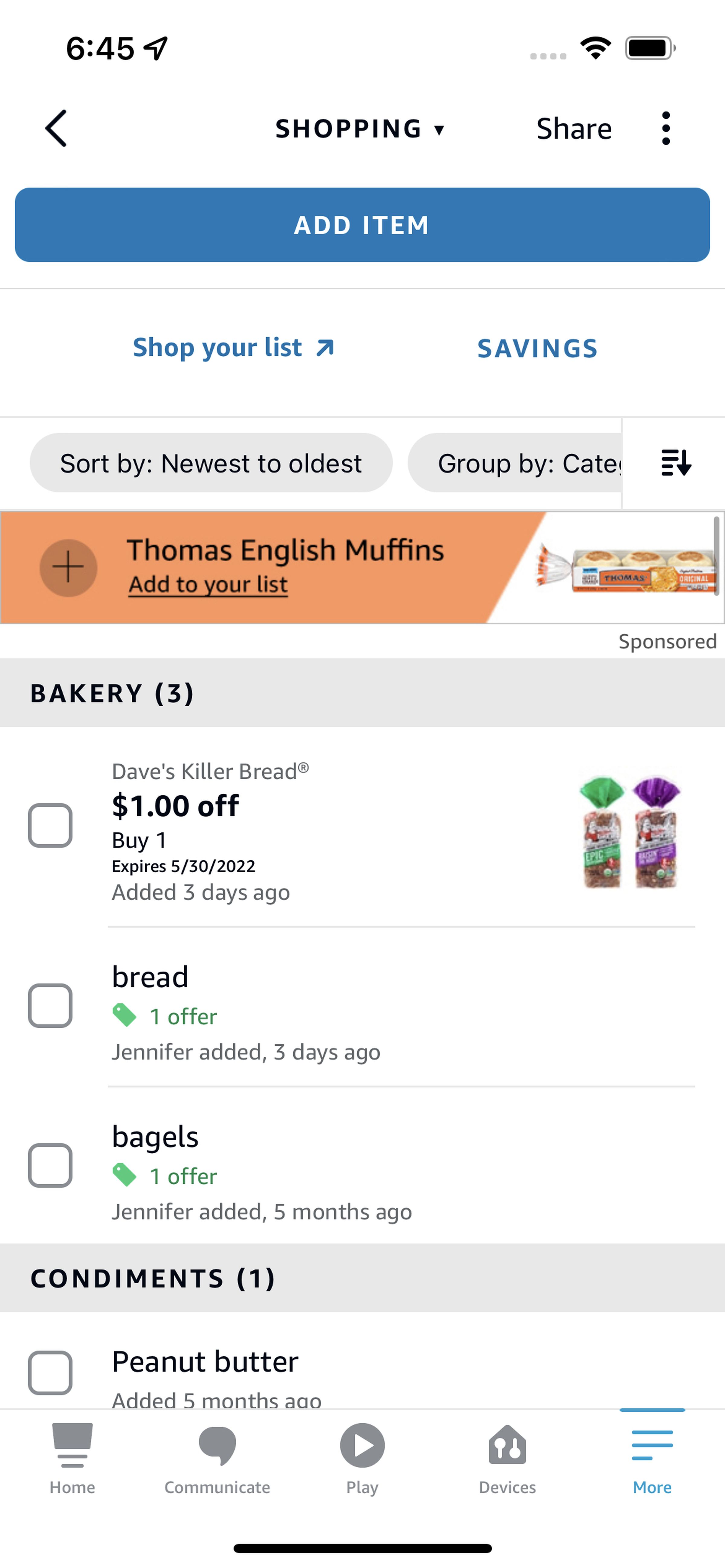The image is a screenshot taken from a mobile device showcasing a shopping application. The status bar at the top shows the time as 6:45, location services enabled, full Wi-Fi signal, but no carrier signal, and the battery nearly full. The user is browsing a shopping website, indicated by a dropdown caret next to the site name, a left-pointing arrow, and a share button. There's a prominent blue "Add Item" button, and a "Shop Your List" feature highlighted in blue, along with a "Savings" section also in blue. 

Users can sort items by newest to oldest. At the top of the shopping list, there is a sponsored post for Thomas' English Muffins, displayed with an orange and white package. Categories listed include "Bakery" with three items in brackets. There is a specific offer for Dave's Killer Bread, showing a $1 discount on purchases made by May 30, 2022. Two packages of Dave’s Killer Bread are shown in green and purple packaging. 

Green indicators suggest current offers on bread and bagels, and there are also listings for peanut butter and condiments.